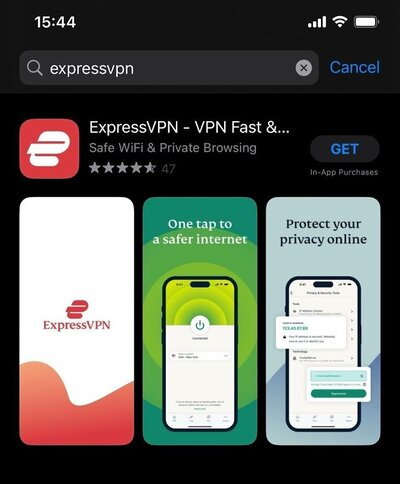The image is a screenshot from a mobile device, potentially a tablet or smartphone, evident from the visible time display (15:44) and the fully charged battery, Wi-Fi, and wireless signal icons at the top corners. The interface appears to be in night mode, featuring a predominantly black background with white text. The content displayed is a section of an app store, likely the Apple App Store.

In the center of the screenshot, a search box contains the text "ExpressVPN." To the right of the search box are an 'X' for clearing the search and a blue "Cancel" button. Below the search bar, an icon with the ExpressVPN logo is displayed, followed by the app's name, "ExpressVPN - VPN Fast Safe Wi-Fi & Private Browsing," and a rating of 47 stars.

A prominent black button with blue text that reads "Get" indicates the option to download the application. The screenshot also features three preview images of the app. The first image bears the title "ExpressVPN," the second image displays the text "One tap to a safer internet," showing a phone interface of the app's functionality, and the third image states "Protect your privacy online," also displaying a phone interface with various application buttons.

The overall theme of the screenshot conveys an emphasis on security and privacy, highlighting the features and user interface of the ExpressVPN application.